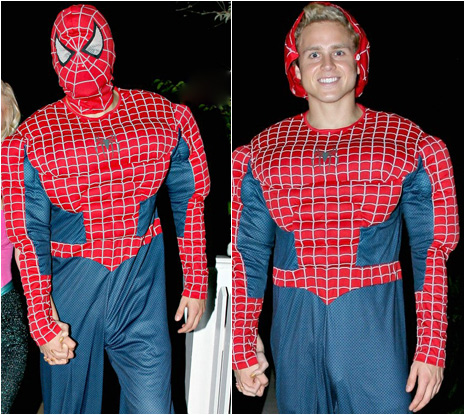The image features two photos side by side. On the left, a person dressed in a classic red and blue Spider-Man costume stands confidently. On the right, the same individual, who appears to be Spencer Pratt from the early 2000s MTV reality show "The Hills," has removed his Spider-Man mask, revealing his smiling face and distinctive blonde hair. Spencer is holding hands with someone whose hand is not fully visible in the frame. The background in both images is uniformly black, highlighting the contrast between the costumed and unmasked versions of Spencer.